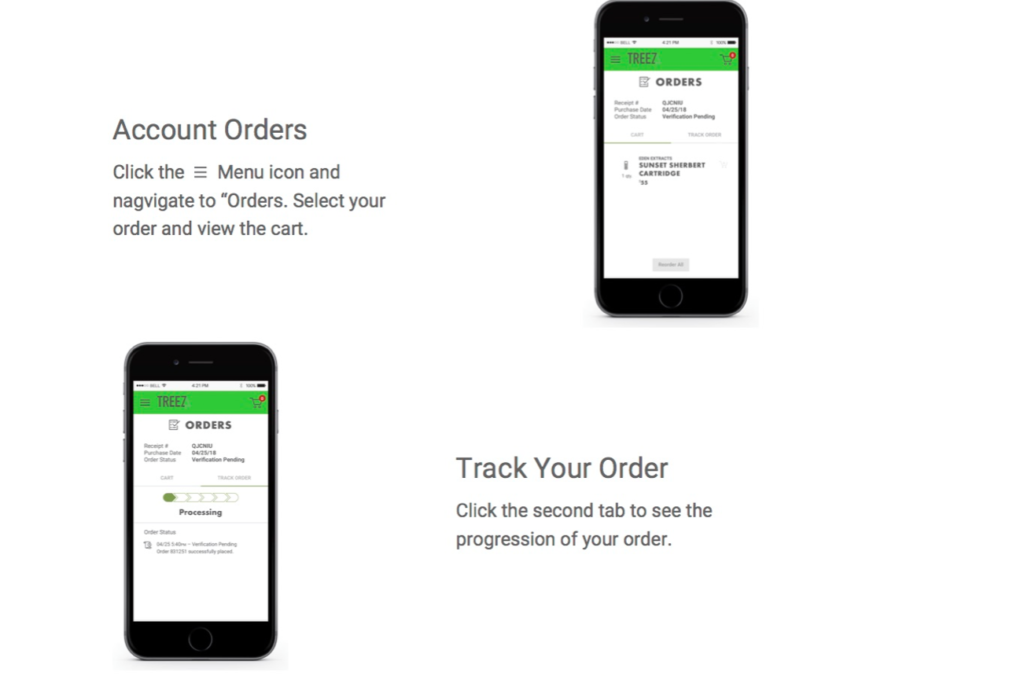The image appears to be a mock-up demonstrating the user interface of a mobile app. In the top left corner, it displays the text: "Account Orders." Below this, there are instructions: "Click the menu icon (three bars) and navigate to Orders. Select your order and view the cart." To the right of this text, a smartphone screen is depicted, reflecting the described interface. On the phone's screen, the text "Trees" (stylized with a 'Z') is visible in the top right, while a cart icon occupies the top left corner. The bottom half of the image features the phone on the left side, displaying an order being processed. Adjacent to this, the right side of the image instructs users: "Track Your Order. Click the second tab to see the progression of your order." All text within the image is presented in a gray color, complementing the overall guide for using the app’s order tracking feature.